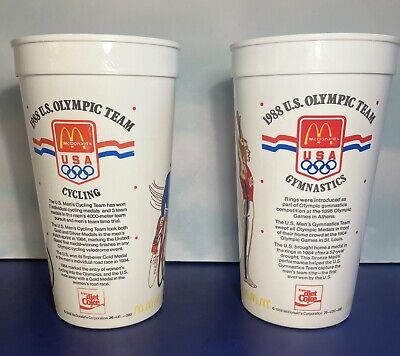This image features two commemorative plastic cups from McDonald's celebrating the 1988 U.S. Olympic team, specifically the gymnastics and cycling teams. The cups prominently display both the Olympic Games and McDonald's logos. The design on each cup includes graphics depicting an athlete relevant to each sport—one cup shows a gymnast with arms stretched out, while the other features a cyclist in motion. The text on the cups, though hard to read due to blurriness, likely provides information about the teams or athletes. The background is a mix of white and blue, and the cups also include a red, white, and blue motif, somewhat reminiscent of the U.S. flag, enhancing the patriotic theme.